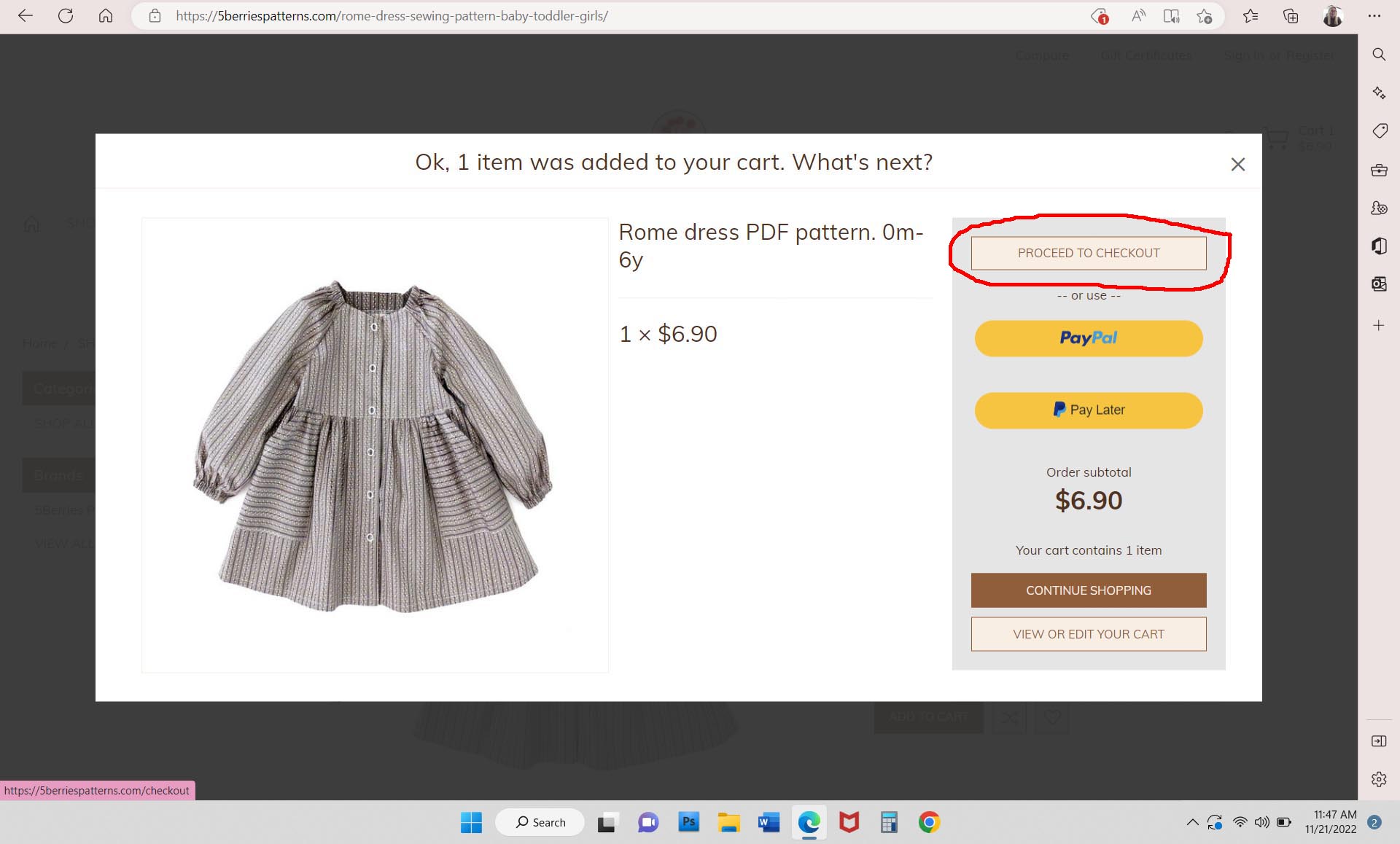A person is browsing an online shopping website in this image. The webpage is surrounded by a light gray border, approximately half an inch thick, along the top, right side, and bottom. Along the top of the border, starting from the left, there is a black left-pointing arrow, a black refresh icon, and a black home icon. Adjacent to these icons is a search bar that nearly spans across the right side. The URL displayed in the search bar is "https://5berriespatterns.com/roam-dress-sewing-pattern-baby-toddler-girls/". At the right end of the search bar, there are four icons followed by three dots, a profile picture, and two additional icons.

Along the right side of the border, there are six vertically aligned icons typically associated with shopping, search, tags, and availability. Behind the central content, the website background appears in a dark grayish hue, but a white pop-up tab occupies the center of the screen. The pop-up message reads, "Okay, one item was added to your cart. What's next?" in black text, with a black 'X' at the top-right corner indicating a close button.

Below this message, to the left, there is an image of a baby outfit with long sleeves. Adjacent to the outfit image, black text reads, "Roam Dress PDF Pattern." Under this, "1 × $6.90" is noted. To the right of this description is a blue rectangular button with "Proceed to Checkout" written in black text, encircled by a red outline. Below this, there are further options in black text: "or use," followed by yellow tabs labeled "PayPal" and "PayPal Pay Later."

The summary section lists "Order subtotal: $6.90" followed by "Your cart contains one item." Beneath this, there is a brown tab with "Continue Shopping" written in white text, and below that, a white tab with "View or Edit Your Cart" written in brown text.

At the bottom of the page is another search bar accompanied by about seven icons. The bottom left corner of the webpage displays the time, date, battery status, Wi-Fi signal strength, and volume level.